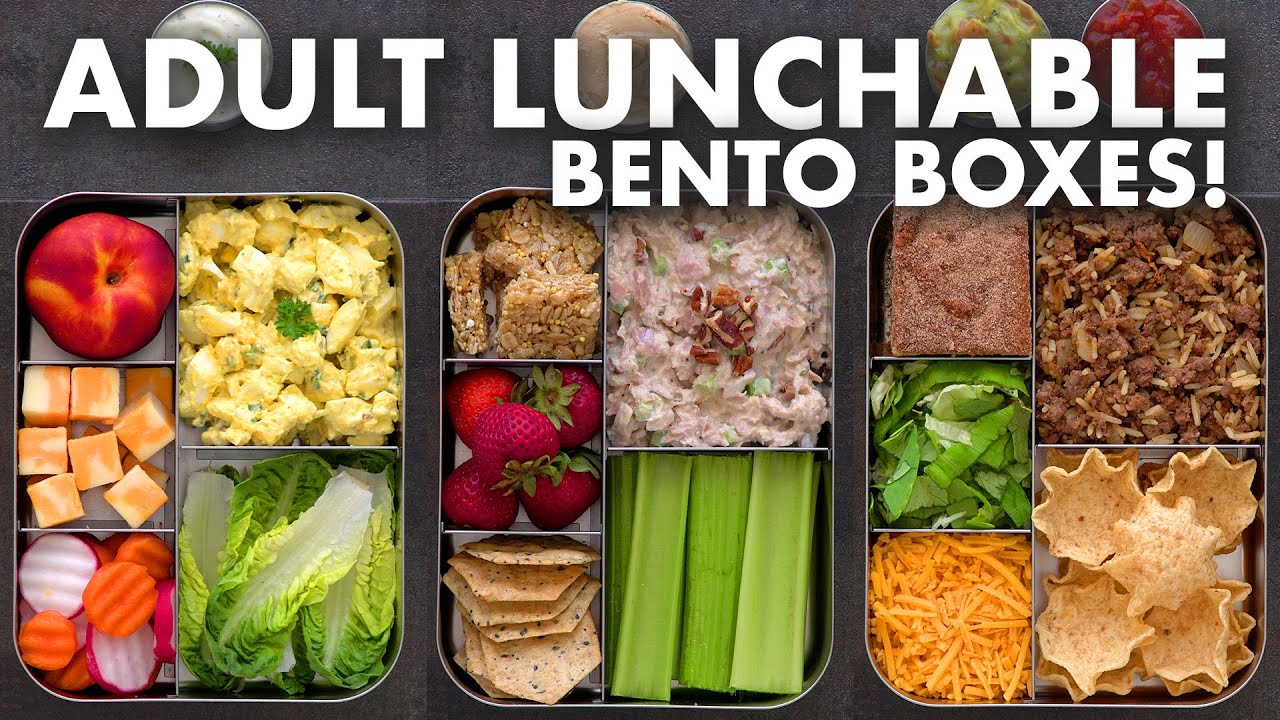The image features three distinct food trays, each labeled as "Adult Lunchable Bento Boxes." 

In the first tray, there are five compartments. One compartment holds a fresh nectarine, another has chunks of cheese. The next section contains peeled carrot and radish slices. The fourth compartment appears to hold a chicken salad, while the final section is filled with various types of lettuce.

The second tray also has five compartments. It includes a granola-type cookie snack, fresh strawberries, and pita chips. One section contains either tuna fish or chicken salad, and the last compartment has celery sticks.

The third tray features five more sections: one contains a piece of coffee bread, another has a fresh salad. There is also a section with cheese, another with taco meat, and the final compartment holds scoopable corn chips.